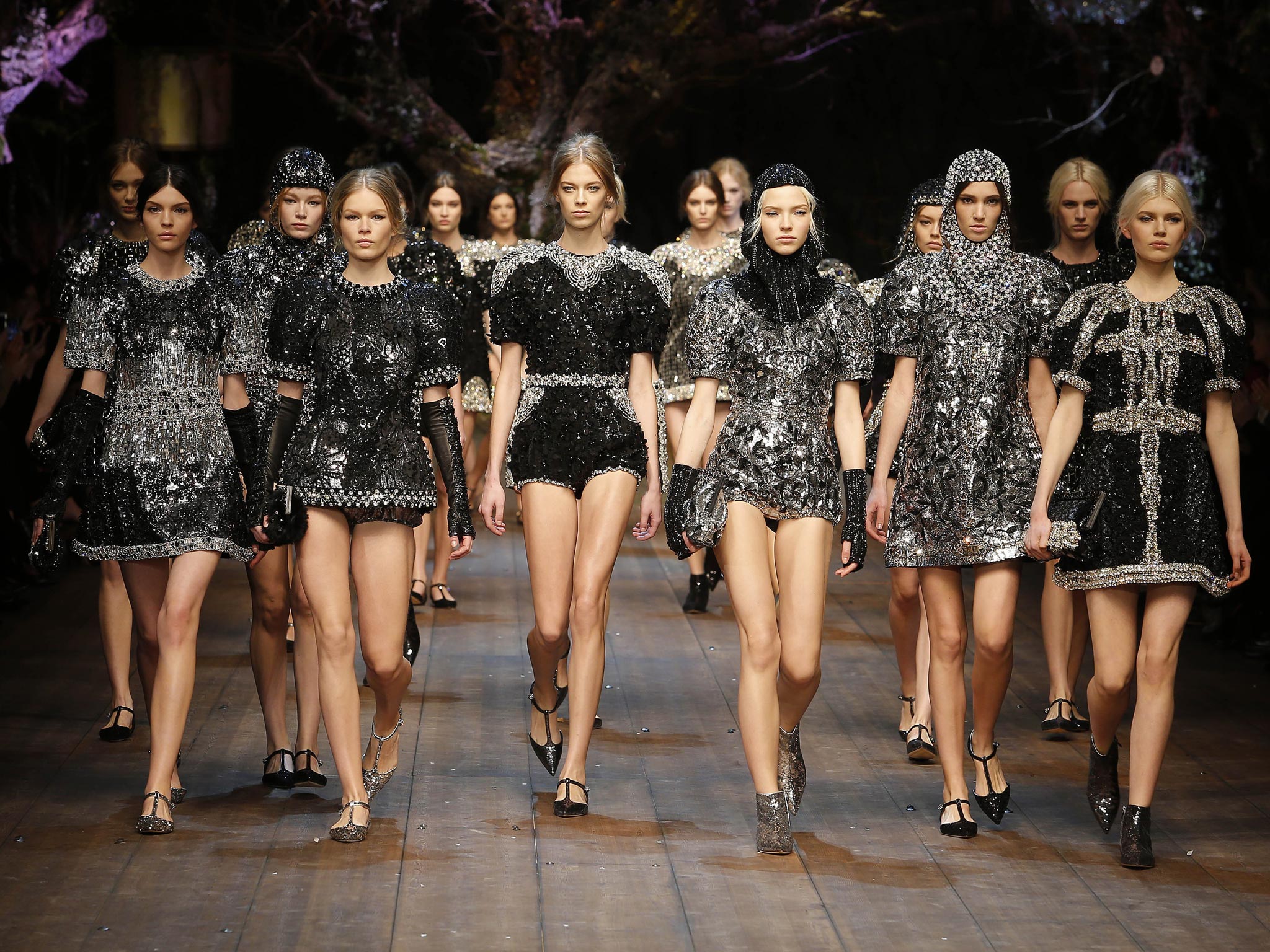A striking group of at least 15 runway models, predominantly white women, stride purposefully towards the viewer in a coordinated fashion. The models are arranged in two rows: approximately five in the back and around ten in the front. They all don outfits comprising either entirely black or a combination of black and silver, with many featuring intricate chain mail-like decorations around the shoulders and chest. The clothing is notably short, ranging from very short skirts to short shorts, revealing their long, slender legs. Each model sports high heels, either black or gray. Some of the outfits are adorned with small silver dots, adding a touch of sparkle to their already eye-catching ensembles. The central figure, one of the taller models, wears a particularly striking black dress with a high hemline and silver accents on the shoulders and chest. The runway is set against a minimalistic black background, with a light brown floor beneath their feet, enhancing the contrast and spotlighting the models. The overall scene exudes elegance and coordination, presenting a captivating fashion moment.